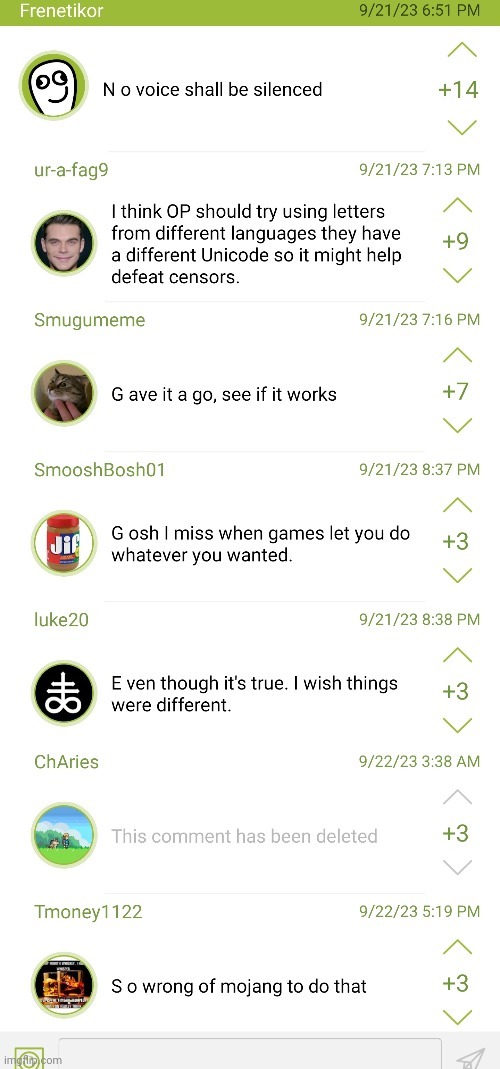A detailed descriptive caption for the image could be:

"A screenshot of a message board dedicated to gaming discussions is displayed. The interface features an olive-green header banner at the top, which includes the text 'Frenette to Core' on the left side and a date and time from the year 2023 in the evening on the right side. Below this banner, numerous comments are arranged in rows. Each comment is preceded by an avatar or icon with the commenter’s name underneath, followed by their brief comment. On the right side of each comment row, there are up and down arrows indicating numerical values, representing user votes or likes. All the numeric values displayed in these voting indicators are positive."